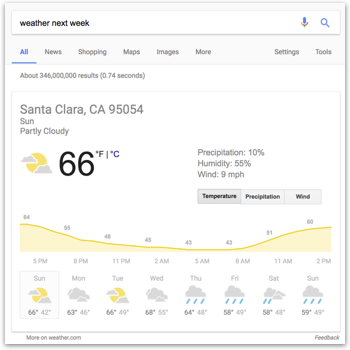The image depicts a detailed weather report screenshot. At the top, there is a gray background with a rectangular white search bar containing the text "weather next week", flanked by a microphone icon and a magnifying glass icon. Below the search bar, navigation options are displayed, including "All," "News," "Shopping," "Maps," "Images," "More," "Settings," and "Tools," with "All" highlighted in blue and underscored with a blue line.

The search results indicate approximately 346 million results found in 0.74 seconds. Beneath this, a boxed weather update is presented, bordered in light gray and having a white background. This section shows the weather for Santa Clara, California, 95054, reporting partly cloudy conditions at 66°F, with 10% precipitation probability, 55% humidity, and current winds at 9 miles per hour.

Further down, three gray boxes titled "Temperature," "Precipitation," and "Wind" provide more details. Additionally, there is a graph featuring a yellow line indicating temperature trends, which starts high, dips, and then rises again towards the end. Below this, a seven-day forecast is displayed, predicting rain for four consecutive days at the end of the upcoming week.